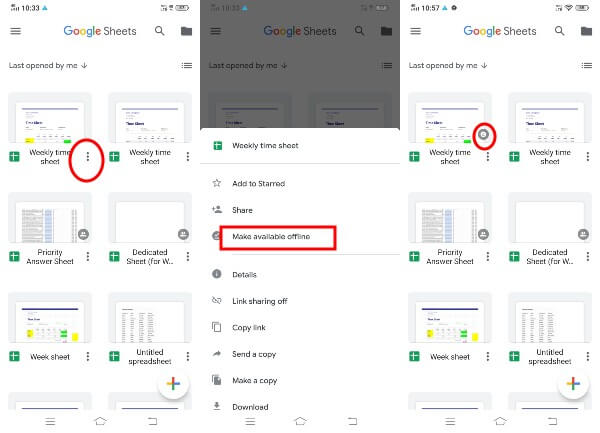The image consists of three side-by-side screenshots of Google Sheets web pages as viewed on cell phones. The screenshot in the center displays the Google Sheets interface with a noticeable gray square obscuring the Google Sheets logo at the top of the page. Several elements are highlighted: one circle highlights the three-dot dropdown menu, which allows users to manage their Google Sheets with options to open, delete, share, or download a file. In this instance, the highlighted option is "Make available offline," indicating the sheet can be downloaded for offline use. The screenshot on the right features a highlighted icon within the thumbnail, signifying that the Google Sheet has been successfully made available for offline access. This means the sheet can be viewed without an internet connection, provided the Google Sheets app is installed on the device.